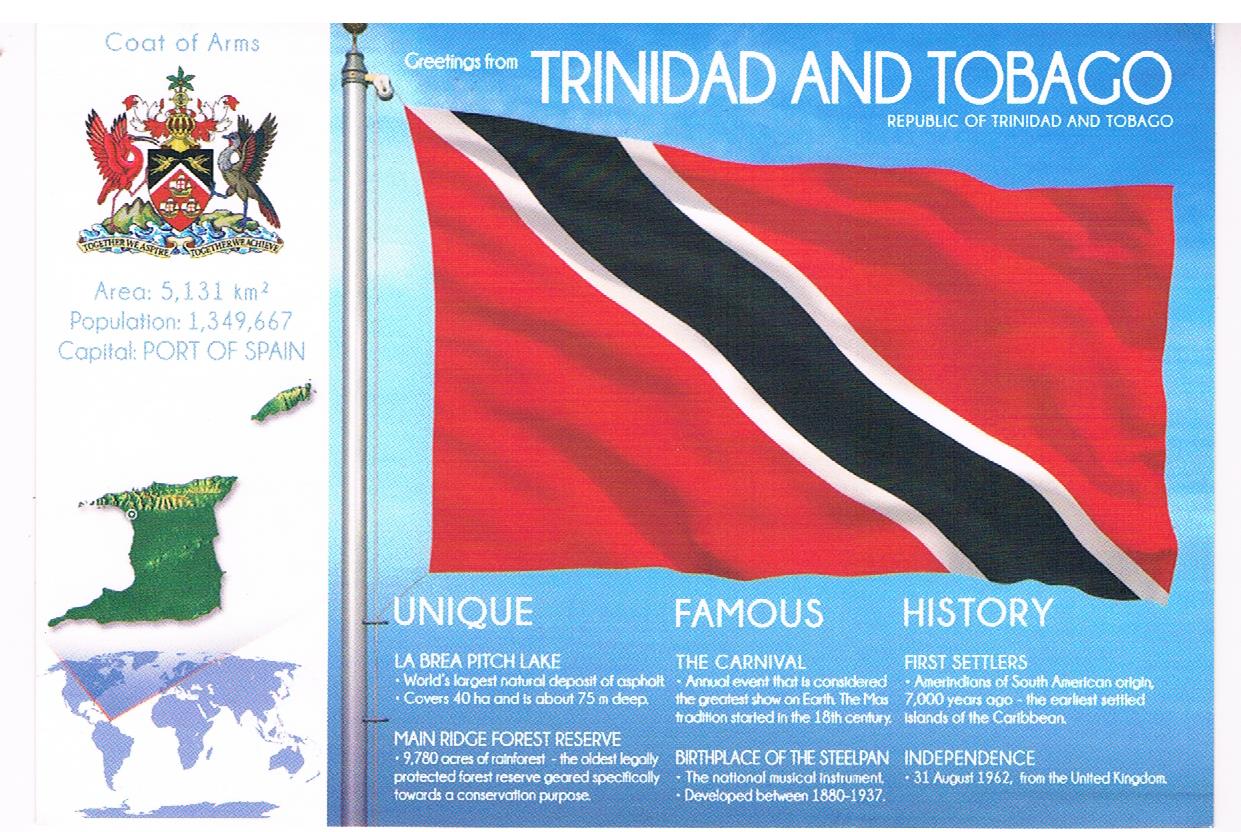This image resembles a colorful and informative postcard from Trinidad and Tobago, seemingly scanned from a magazine. Dominating the left side is a white vertical rectangle featuring the nation's coat of arms. This coat of arms showcases two vibrant birds, one red and one black, perched on either side of an ornate shield, symbolizing the country's rich heritage. Below the coat of arms, the postcard lists essential statistics: an area of 5,131 square kilometers, a population of 1,349,667, and the capital, Port of Spain. Adjacent to these details are a satellite image and a geographical map pinpointing the location of Trinidad and Tobago in the Caribbean.

To the right of this informational column, the postcard proudly displays the flag of Trinidad and Tobago. Waving against a serene blue sky, the flag is striking with its red background bisected diagonally by a bold black stripe bordered by thin white stripes on each side. Above the flag, the text reads "Greetings from Trinidad and Tobago, Republic of Trinidad and Tobago," while below it, the caption "unique famous history" hints at the island's rich cultural tapestry. Historical insights include mentions of the first settlers from South America and notable landmarks such as La Brea Pitch Lake, the world's largest natural asphalt deposit, and Trinidad and Tobago's distinction as the birthplace of the steel pan.